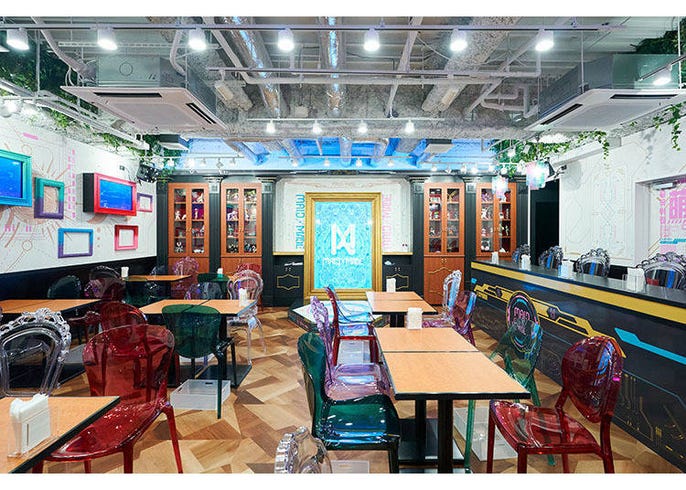This is a color photograph of a vibrant and modern indoor space, likely a restaurant or bar. The floor is polished wood parquet, and the seating consists of wooden four-top tables accompanied by transparent lucite chairs in a variety of colors, including green, clear, red, and purple. The scene features an industrial-style ceiling, complete with exposed pipes, ductwork, and multiple track lighting arrangements that brightly illuminate the area.

On the left side of the room, a white wall is adorned with variously shaped and colored picture frames, seemingly empty. The back wall, painted a dark charcoal gray, houses built-in cabinets with glass doors. Though objects can be seen inside these cabinets, their details aren't discernible. A notable feature is a light blue picture within a large gold frame situated on this wall. 

To the right, there is a long black bar with additional tables and chairs on the opposite side, notable for the absence of seating right in front. Beyond the bar, four chairs are visible. The setting includes a space that might be an entrance, marked by a door or window displaying an emblem resembling a cross. Overall, this well-lit environment exudes a contemporary and eclectic atmosphere, perfect for social gatherings.